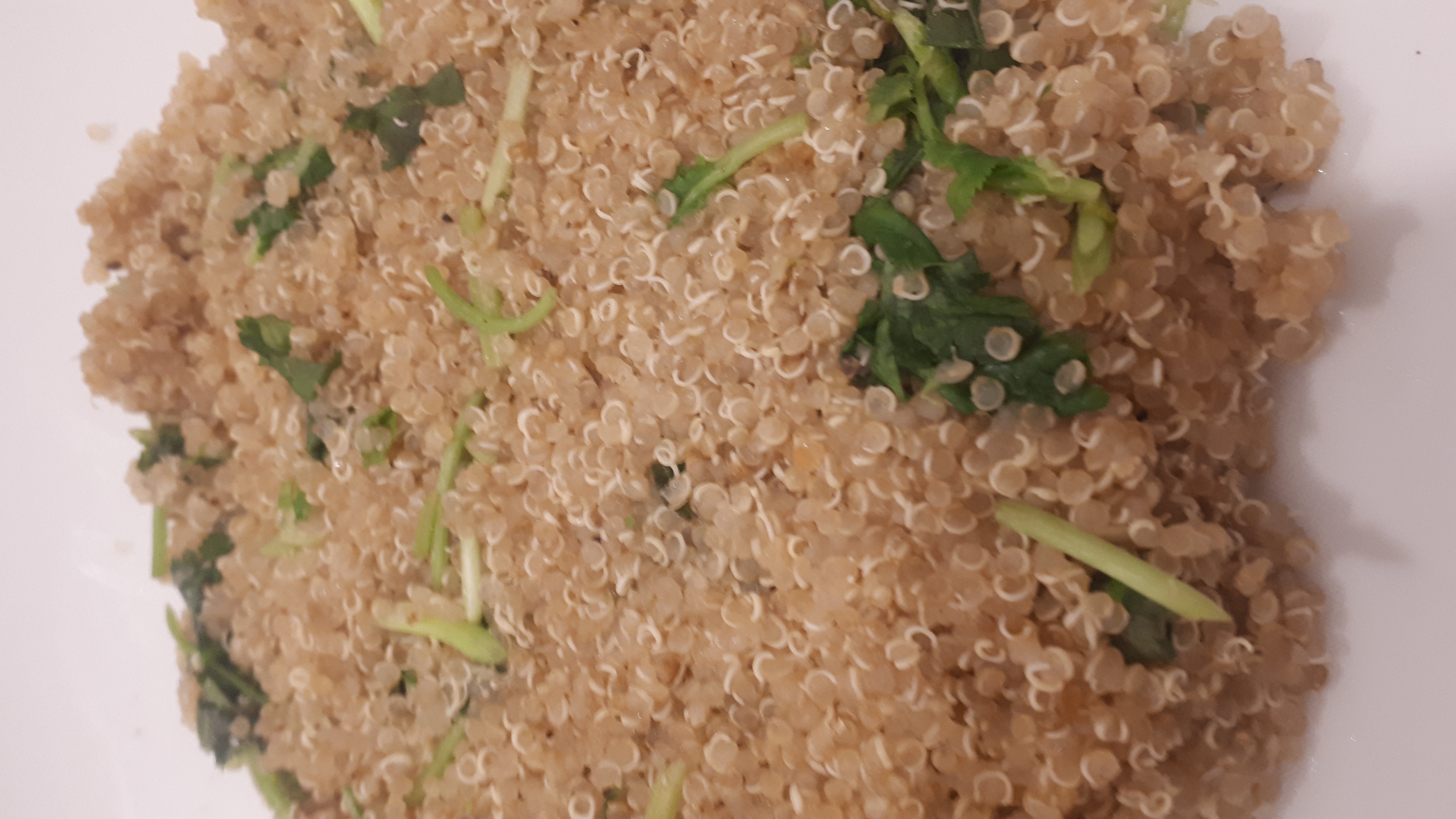This close-up image features a generous, cake-style serving of cooked quinoa, positioned against a white background with no visible dish. The fluffy, light brown quinoa has a slightly darker brown edging, and its fibrous texture is characterized by separated grains and stringy white bits. Mixed into the quinoa are small, torn pieces of green onion, ranging from light to dark green, with the darker green pieces appearing more leafy. The serving, resembling a thick, round cake, looks substantial enough to be a filling meal.